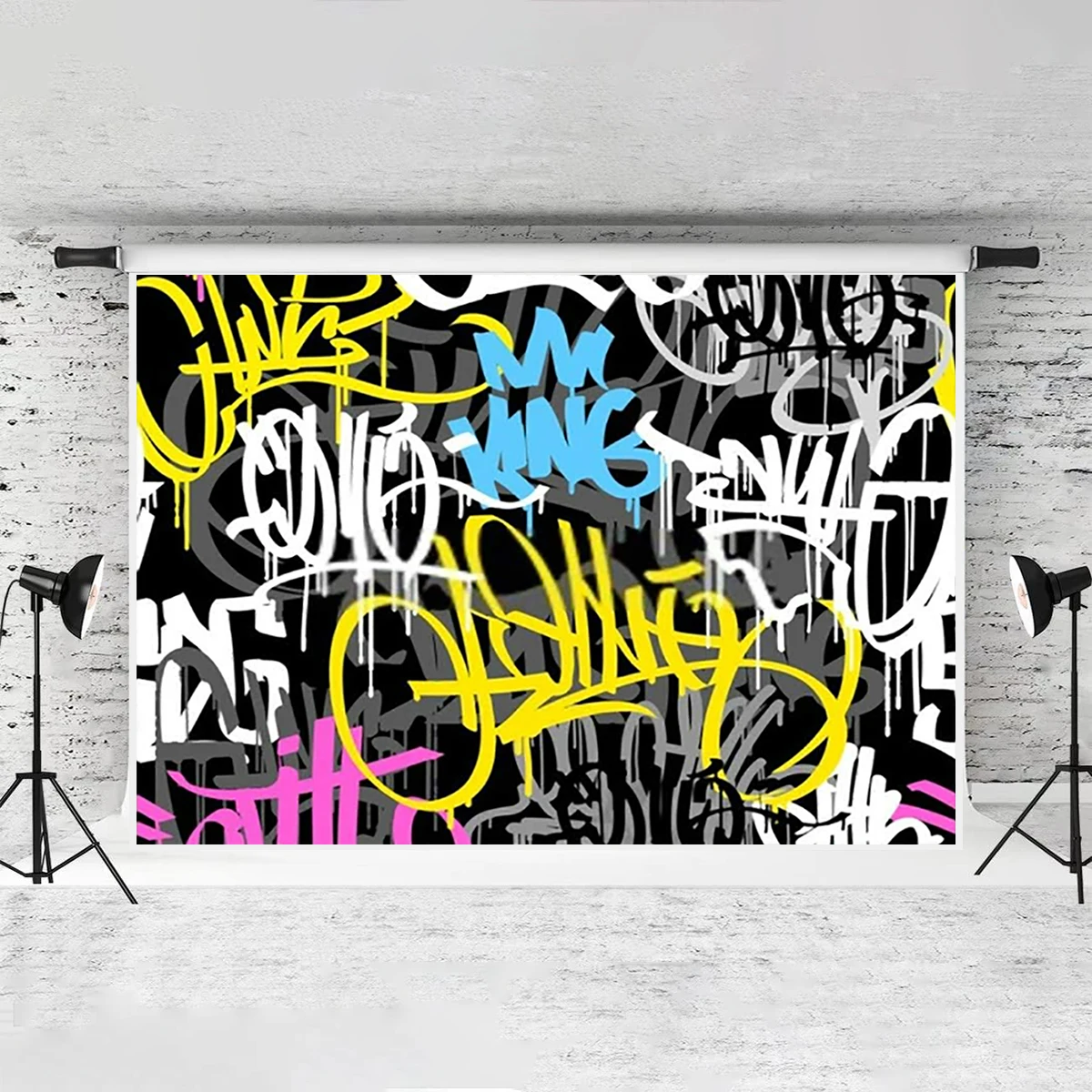The image is a computer-generated depiction of a piece of graffiti art set against a white brick wall. This digitally rendered artwork showcases a white canvas with a black background, covered in a vibrant mix of graffiti. The graffiti is composed of abstract squiggles and shapes, incorporating colors such as white, black, gray, bright yellow, and bright pink. At the center, clearly readable in bright blue, are the words "My King". Beside the blue inscription, there are additional abstract letter-like forms in pink and yellow, some of which appear to be dripping paint. The artwork itself is displayed as if it were a print hanging from a roller, akin to a pull-down screen at a movie theater. Flanking the graffiti art are two large, black spotlights with metal stands and shades, positioned on either side to illuminate the vibrant piece. The floor beneath appears gray, complementing the overall urban aesthetic of the scene.